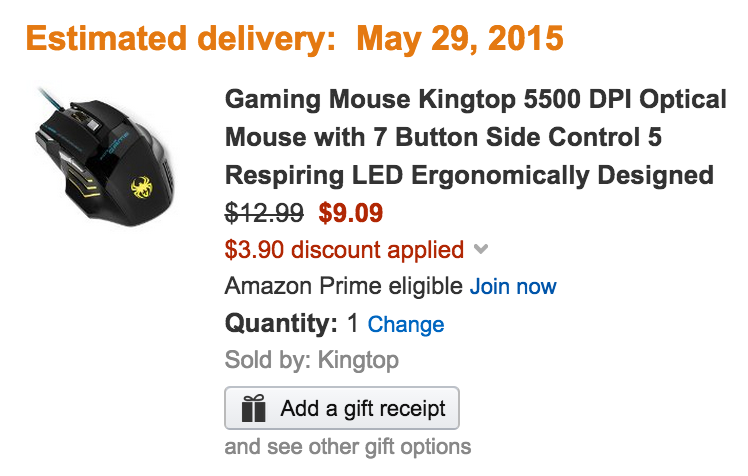The image appears to be a confirmation screen following a purchase on Amazon, dated with an estimated delivery of May 29, 2015, prominently displayed at the top in orange letters. The main focus is an image of a sleek black computer mouse adorned with a striking yellow spider design. Beneath the image, the product description is detailed in black letters: "Gaming Mouse, Kingtop 5500 DPI Optical Mouse with 7 Button Side Control, 5 Respiring LED, Ergonomically Designed."

Originally priced at $12.99, the new price is reflected as $9.09 in bold red numbers, indicating a $3.90 discount. This price adjustment is highlighted with a red strikethrough of the original price. Below the price, a grey downward arrow directs attention to further details stating "Amazon Prime eligible," with a prompt in blue letters "Join now."

Continuing downwards, the quantity is specified as "1" in dark black type, accompanied by an option to "Change" in blue letters. Further below, it notes in gray letters that the item is "Sold by Kingtop." The bottom section of the screen features a rectangle with a gift package icon, offering options to "Add a gift receipt" and "See other gift options."